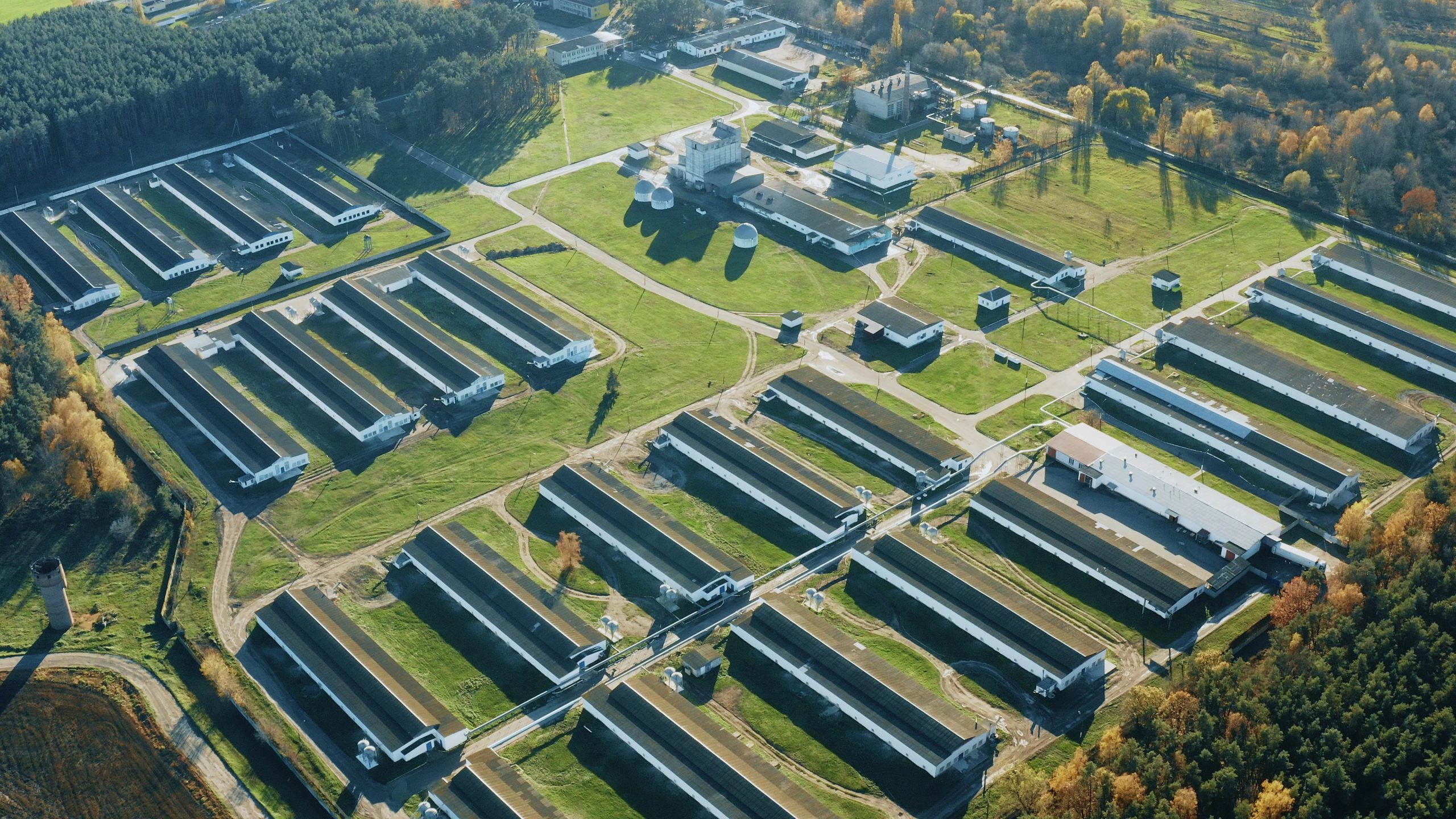This aerial photograph showcases a large, organized facility with numerous similarly designed rectangular buildings. Each structure features a dark roof, either brown or black, with a white outline and white-painted siding. The buildings are arranged in neat rows, specifically forming four distinct lines. The surrounding environment includes well-maintained green grass fields and light-colored paths, likely roads, that provide access to the buildings. Notably, there's a concentration of circular structures in the central part of the facility. To the right, a standout building possesses a different white-colored roof. Additional buildings and possibly a factory can be seen further in the distance. The entire scene is bordered by green and gold trees, adding a natural perimeter to the area. This image provides a detailed view of a meticulously organized compound, possibly industrial or agricultural in nature.